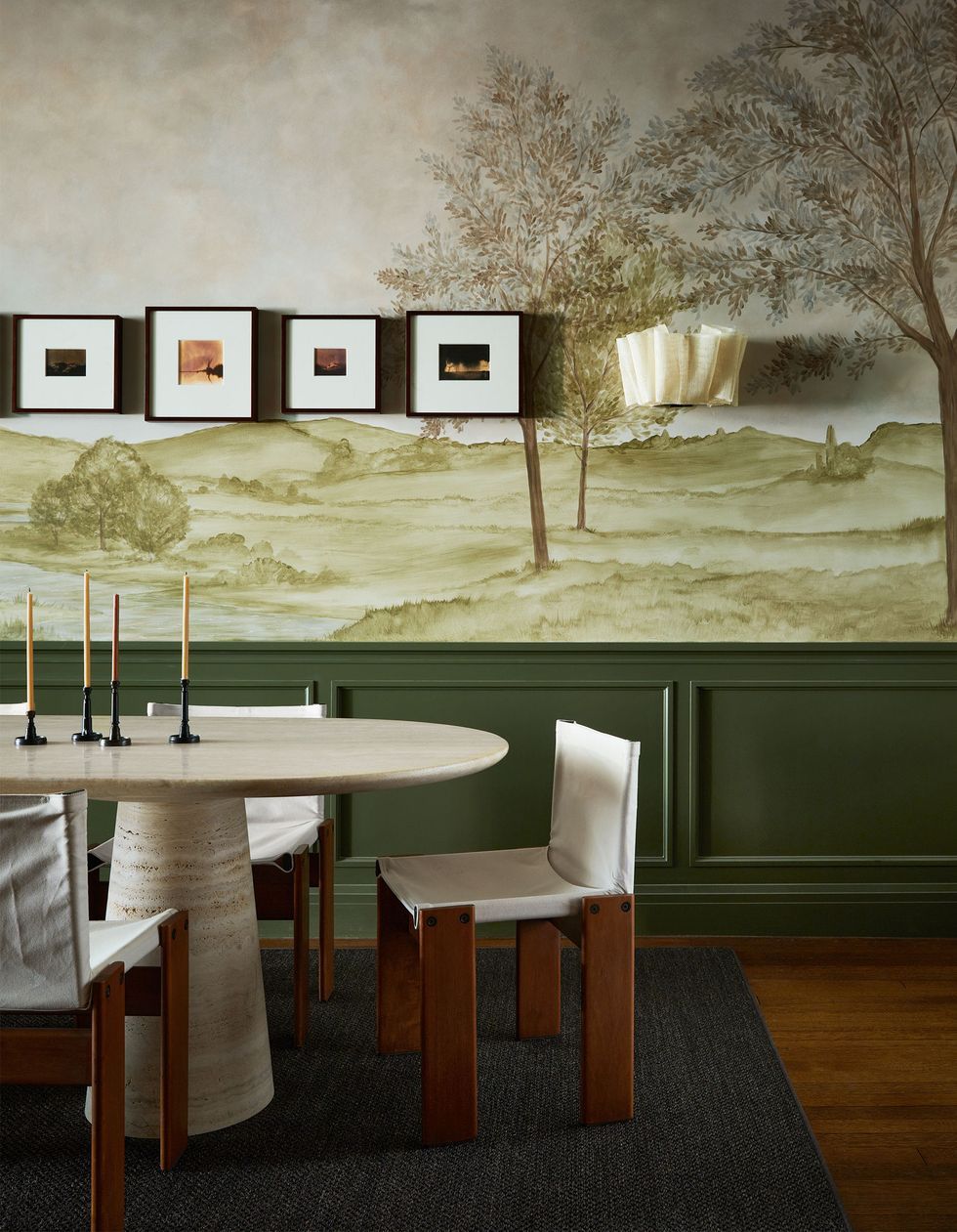The image depicts a dining space with a blend of modern and natural elements. The focal point of the room is a sleek, oval-shaped dining table with a columnar cone-like base. The table, which appears to be a light slate gray, is adorned with four pillar candles on green candlesticks, adding a touch of elegance. Surrounding the table are three chairs featuring brown wooden legs and white canvas seats and backs, creating a clean, minimalist aesthetic.

The floor is covered with brown wooden slats, and a gray rug defines the dining area. The backdrop of the room is particularly striking with its dual-tone wall design. The upper portion of the wall features wallpaper depicting a serene green field scene with trees, shrubs, and rolling hills. Below the wallpaper, the wall is paneled with evergreen-colored wainscoting, providing a rich contrast.

Adorning the wall are four small photographs, each framed in black with white matting. These pieces of artwork add a personal touch to the space. Additionally, there appears to be a small shelf or perhaps a light fixture to the right of the photographs, potentially holding napkins or other small items.

The overall atmosphere of the dining area is one of simplicity and tranquility, harmoniously blending modern furniture with nature-inspired decor, all set against the warmth of a wooden parquet floor.